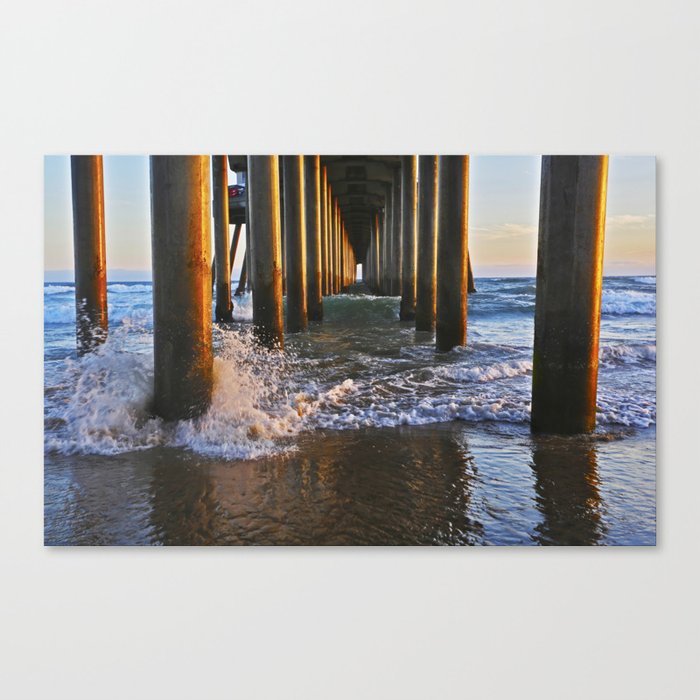This well-composed, professionally taken full-color photograph captures an ethereal scene beneath a pier extending into the ocean. Framed within a square aspect bordered by a thicker top and bottom edge, the image draws the viewer's eye along the symmetry of the wooden pillars, stretching from the shoreline into a distant pinpoint of light, creating a mesmerizing tunnel effect. Captured during the ethereal glow of either sunrise or sunset, the scene is bathed in soft light which illuminates the calm, shallow waters at the foreground. Here, gentle waves crash against the pier's pylons, creating striking contrasts of dark water and white sea foam. A wave on the left is shown splashing halfway up a pylon, highlighting the tranquil yet dynamic interplay between sea and structure. The sky above is mostly clear, painted with subtle hues of yellow and light blue, accentuating the serene ambiance of this coastal moment. The absence of boats and the calm sea enhance the peacefulness of the setting, emphasizing the solitary beauty of the outstretched pier against the rhythmic cadence of the ocean.